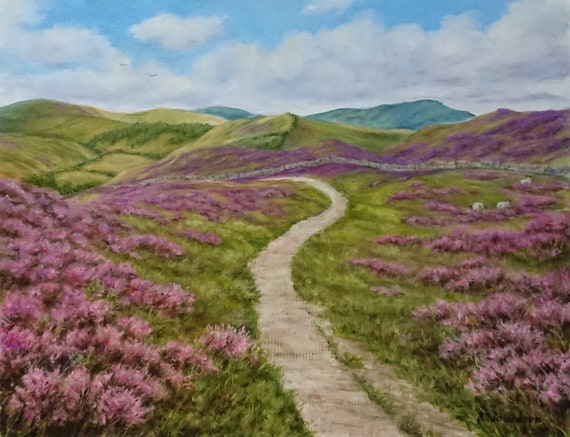This realistic-style painting captures an idyllic outdoor scene featuring a narrow, winding path that threads through a field abundant with purple-flowered plants interspersed with tufts of green grass. The path, gray in color and narrow enough for just one person, starts from the center bottom and meanders through the landscape, disappearing into the middle before looping around a structure reminiscent of Hadrian's Wall—a long, thin stone wall that echoes the surrounding hills' contours. The lower left and right corners of the painting are filled with clusters of vibrant purple flowers.

In the middle section on the right side, three black and white cows graze placidly, adding a touch of pastoral life. The scene is set against a backdrop of gently rolling green hills, which transition to low-lying mountains. These mountains exhibit varying shades of green and blue, enhancing the depth of the landscape, with the most distant mountains tinged blue due to atmospheric perspective. Above this verdant expanse, a blue sky spreads across the top 20% of the painting, adorned with fluffy white clouds and two soaring birds, making the sky feel expansive and alive. The painting is perfectly square in shape, and there is no text present.